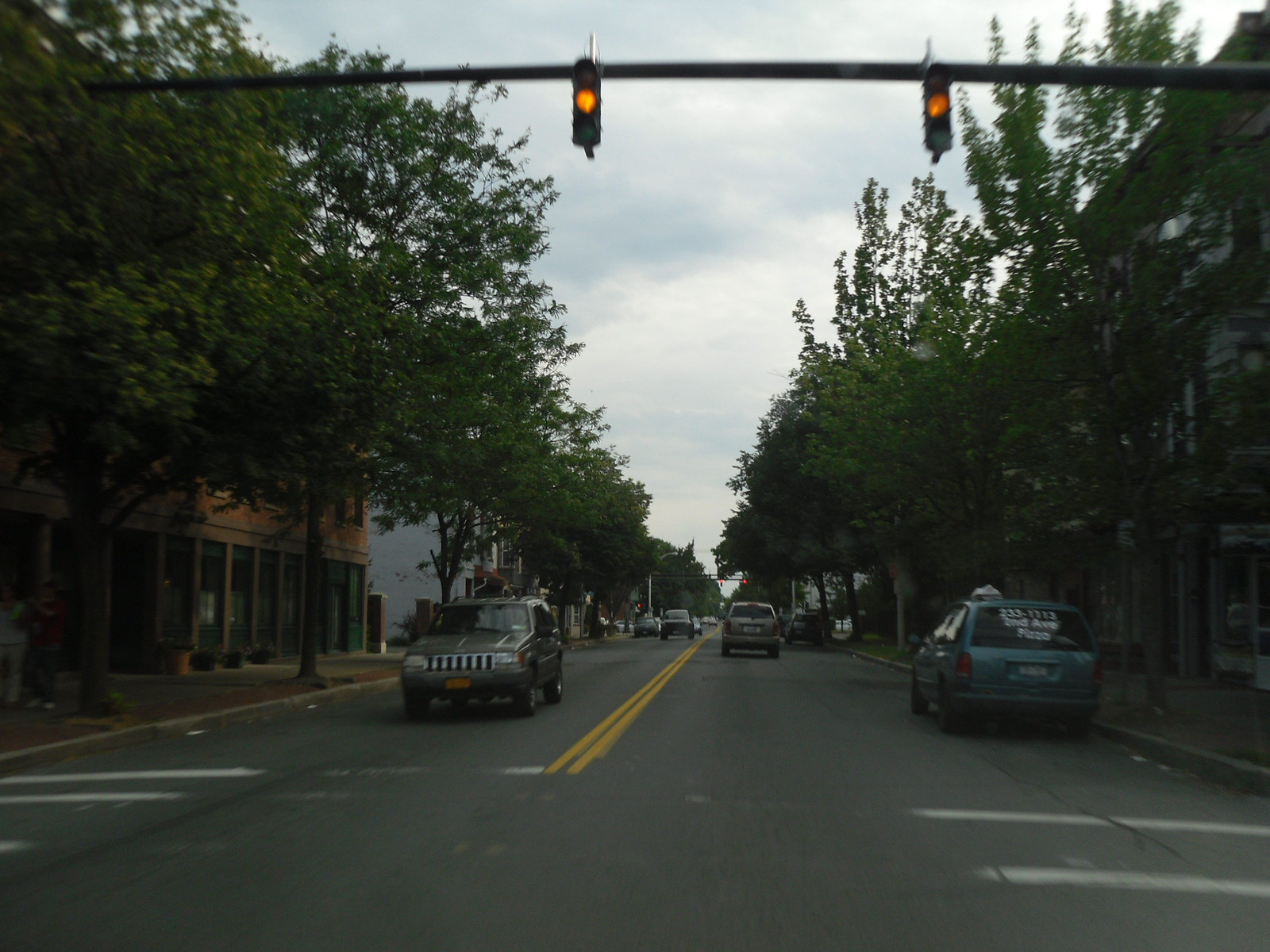This outdoor daytime color photograph, captured in a landscape orientation, presents a detailed city street view. The image, taken from a standing position in the middle of the road, reveals a lane of traffic stretching away from us, with a car visible in the distance traveling away. Starting in the second quarter horizontally, two yellow stripes run from our position down the length of the street, separating the opposing lanes of traffic, typical of North American road markings. The street is bordered by expansive, blooming trees rising from the sidewalks, arching over the buildings that line both sides. These structures appear to be commercial premises, characterized by multiple windows and pillars, indicative of shops or office spaces, rather than residential units. 

The scene includes various vehicles: a blue taxicab parked curbside to the right, a Jeep or SUV waiting at a stoplight facing towards us, and additional cars parked and moving in both directions further down the street. Notably, the stoplights at the top of the image display yellow signals, set against the gray, overcast sky, adding a moody tone to the scene. A faded pedestrian walkway crosses the road, its white lines still discernible near the curb but worn away in the middle. The closest building on the left is a brick structure with numerous windows, suggesting it could be an office or retail shop. Overall, the image captures the essence of a bustling, tree-lined urban street enveloped in a slightly gloomy but detailed atmosphere.